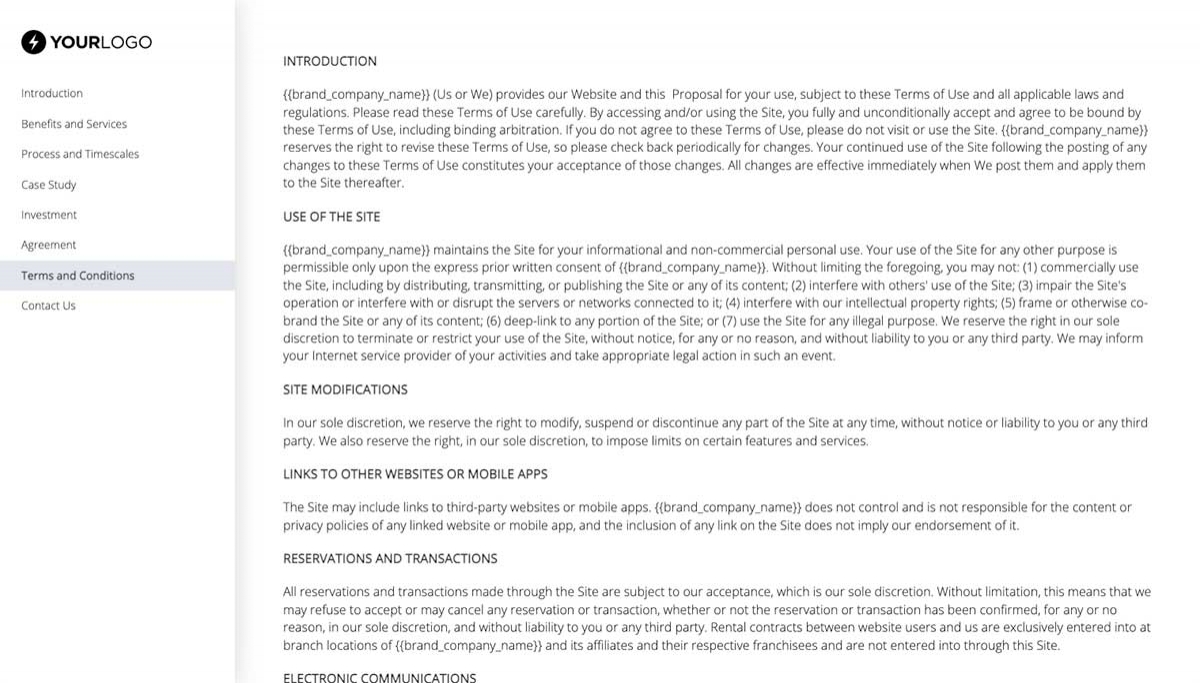The image depicts a stark, minimalist layout of a webpage, characterized by a plain white background and black text. In the top left corner, there's placeholder text that reads "Your Logo," indicating where a company logo should be placed. Adjacent to it, there's a simple icon featuring a white lightning bolt enclosed in a black circle, adding a touch of visual interest to the otherwise basic design.

On the left side of the page, a navigation pane lists several sections: Introduction, Benefits and Services, Process and Timescales, Case Study, Investment, Agreement, and Terms and Conditions. The right side of the page is currently focused on the Terms and Conditions section. The content here starts with an introduction paragraph filled with typical legal language. Throughout, there is generic placeholder text, such as "Your Logo" and "brand_company_name," meant to be replaced with specific information related to the user's company.

The Terms and Conditions cover various legal aspects of using the site, including site modifications, links to other sites, and terms related to reservations and transactions. The overall aesthetic is intentionally plain, reinforcing the straightforward and no-frills presentation of necessary legal details.